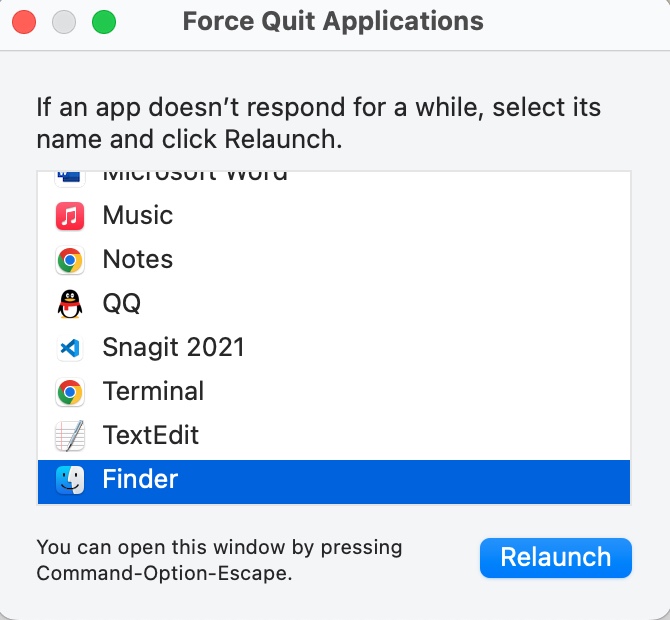The image depicts a "Force Quit Applications" window on a computer screen. The window features a light bluish-gray bar at the top, and a header that reads, "Force Quit Applications." Below this, there is a message: "If an app doesn't respond for a while, select its name and click Relaunch."

On the left side of the window, there are three buttons in a horizontal line: a red button, a gray button, and a green button. The main section lists several applications currently running, each accompanied by an icon. The listed apps are:

1. Microsoft Word
2. Music (represented by a notes icon)
3. QQ (with a penguin icon)
4. Snagit 2021
5. Terminal (accessed through Google, indicated by an appropriate icon)
6. Finder (shown with the traditional Finder face icon)

At the bottom of the window, it instructs users that they can open this window by pressing Command+Option+Escape. To the right of this instruction, there is a "Relaunch" button, which users can click to restart the selected app. This window is typically used to force quit unresponsive applications.